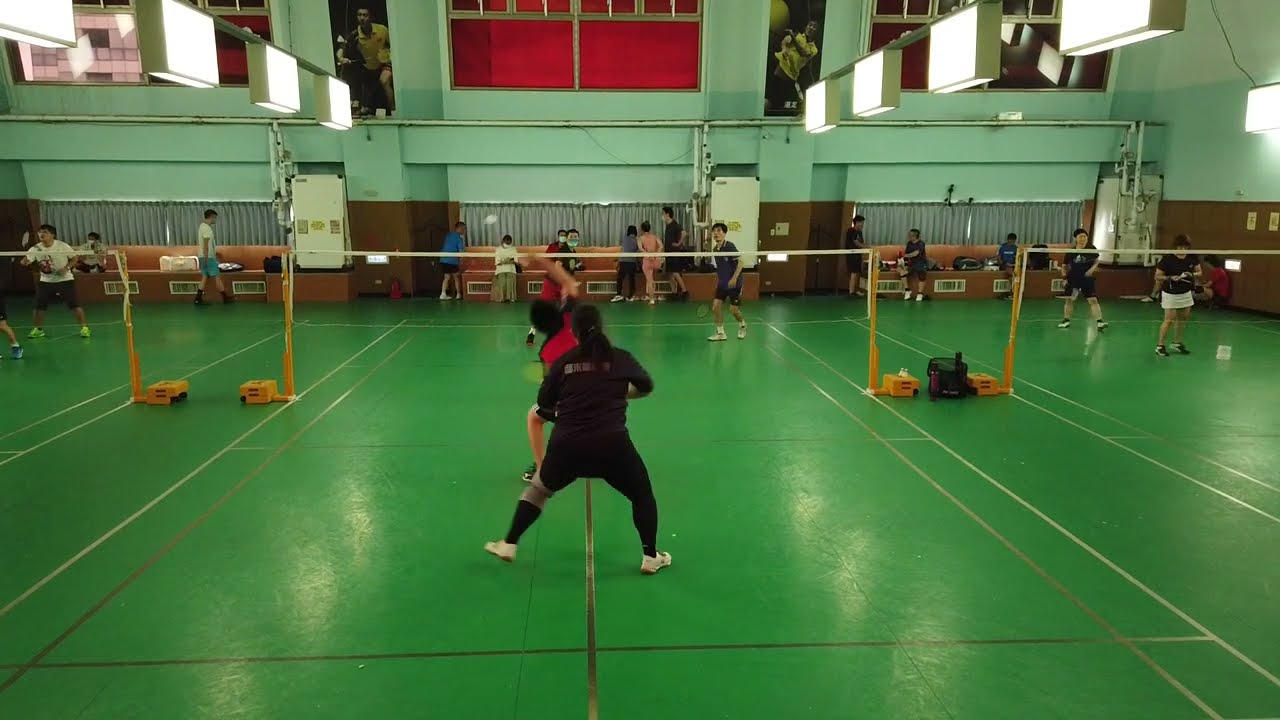The image depicts a spacious indoor scene within a gymnasium, bustling with activity as several games of badminton take place on the green-floored courts. The setup includes at least three playing areas, marked by black and silver lines, with central orange-based nets. The gym walls are lined with brown tables and red curtains, obstructing natural light and creating an ambience illuminated by artistic square ceiling lights. In the middle court, the dynamic action is captured as two teams of two engage in a fast-paced shuttlecock exchange. The players, dressed in athletic gear, appear to be Asian and are actively in motion, making the scene slightly blurry. To the right and left, additional matches are ongoing, with other players evident in various states of preparation, mingling in anticipation of their turn. The background also features booths, posters of badminton or tennis players, and more of the same distinctive ceiling lights, contributing to the vibrant, athletic atmosphere of the indoor sports complex.